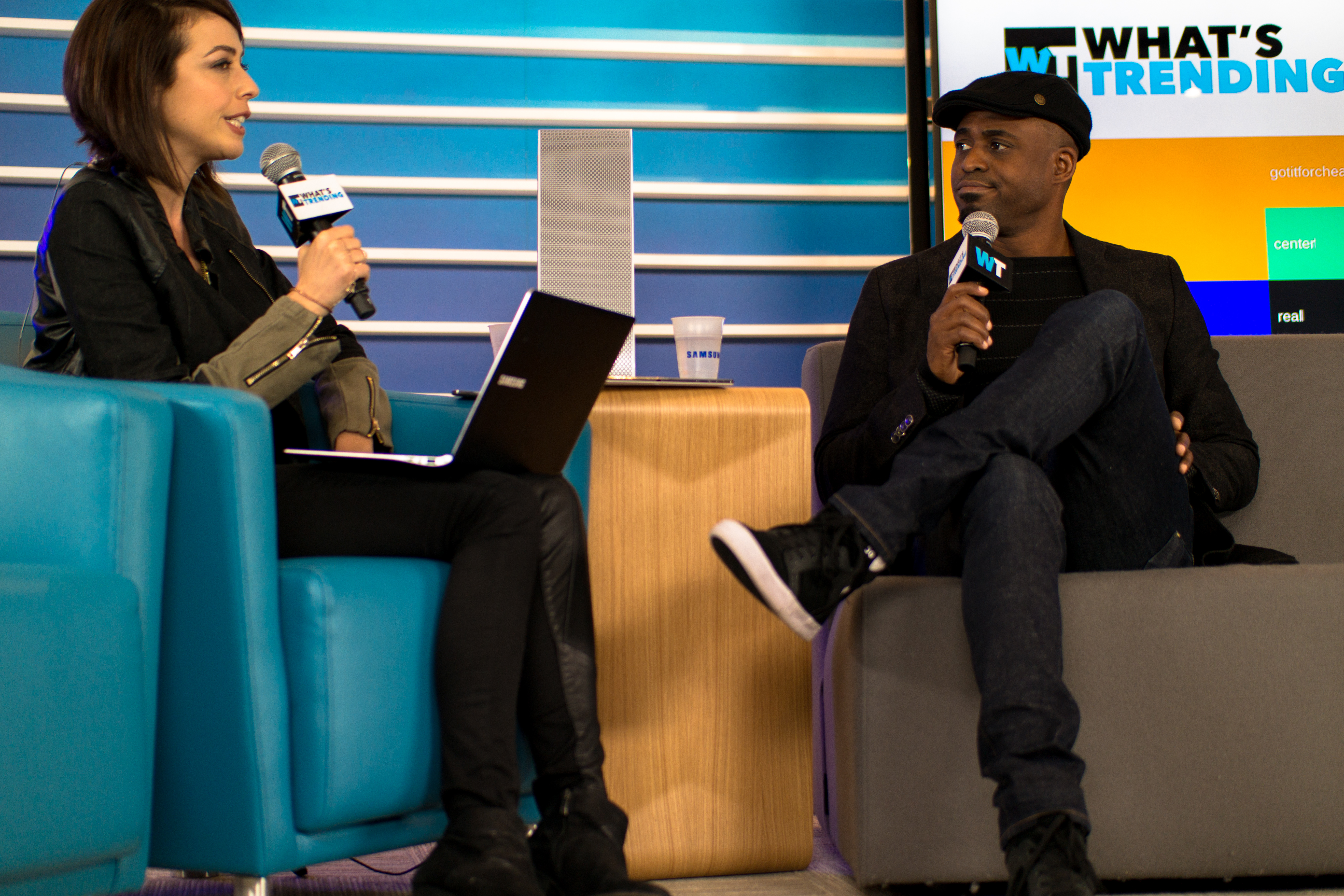In the photograph, two individuals are engaged in a conversation on stage, seated in distinct armchairs. The person on the left, a woman with short dark hair and pale skin, is sitting in a blue upholstered armchair with another empty blue chair beside her. She is dressed in black pants, black shoes, and a black coat with gray sleeves that have zippers partially unzipped. A black laptop with a silver side rests on her lap, and she holds a microphone to her mouth, appearing to speak. To her right, positioned between them, is a slender, light brown wooden side table with a visible wood grain. The table supports a tray with two plastic cups filled with a clear liquid and a speaker. The individual on the right, a dark-skinned man, sits in a gray armchair. He is wearing black pants, black shoes with white soles, a black business coat layered over a black t-shirt, and a black beanie. His left leg is crossed over his right knee, and he too holds a microphone to his mouth. Both appear deep in conversation, with the woman speaking and the man watching her skeptically. The background showcases a mix of blue, white, orange, and teal elements.